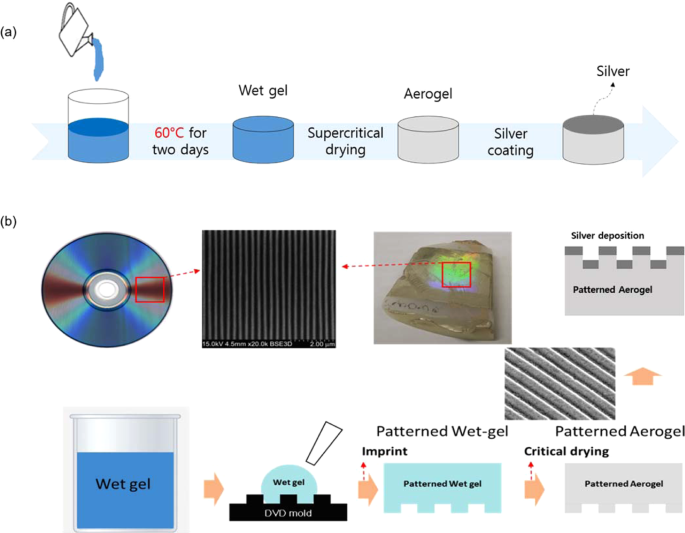The image portrays a detailed step-by-step process of creating a patterned aerogel, essential for certain applications, including CDs. At the top, labeled A, an outlined drawing of a watering can pours blue liquid into a glass cylinder labeled "60 degrees Celsius for two days." This results in a wet gel within the cylinder. Subsequently, the gel undergoes supercritical drying, transforming it into a gray substance referred to as aerogel. The aerogel then receives a silver coating, transitioning into a silver-topped cylinder. Below this, labeled B, the process connects to further stages involving the patterning of aerogel. This involves steps with images including a CD and additional gel manipulations, suggesting the aerogel is patterned and structured further for specific uses, like the fabrication of CDs. The diagram combines visual and textual elements to clearly illustrate the intricate procedure.